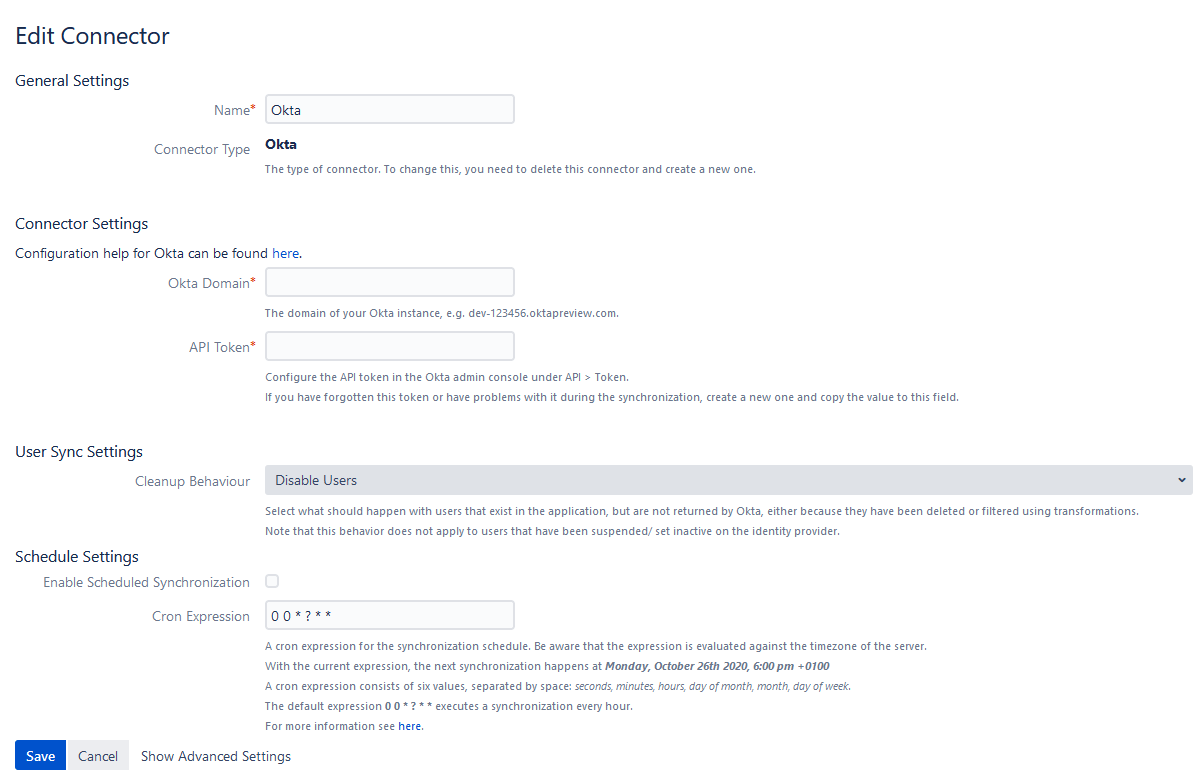The image displays a section of a website interface with the heading "Edit Connector" prominently written in black text against a white background. Under this heading, slightly smaller but still capitalized, is "General Settings." The section contains multiple labeled input fields and settings options.

1. **Name** (with a red asterisk indicating a required field): The input field contains the text "Okta," starting with a capital 'O'.
2. **Connector Type**: This field is filled with "Okta" in bold, dark print. A note follows explaining that to change the connector type, the user must delete the current connector and create a new one.
3. **Connector Settings**: This section provides a hyperlink for assistance with configuration details specific to Okta. 
    - **Okta Domain** (with a red asterisk): An empty input field is provided.
    - **API Token** (also with a red asterisk): Another empty input field follows.

Below these fields, the interface delves into additional settings:
4. **User Sync Settings**:
   - **Cleanup Behavior**: This includes an option labeled "Disable Users," presented within a medium gray banner.

5. **Schedule Settings**:
   - **Enable Schedule Synchronization**: An unchecked box likely intended for enabling this feature.
   - **Cron Expression**: An accompanying input space allows for the entry of a cron expression, accompanied by a description.

At the bottom of the interface, there are options to either "Save" or "Cancel" the changes, along with a link to "Show Advanced Settings" for more detailed configuration.